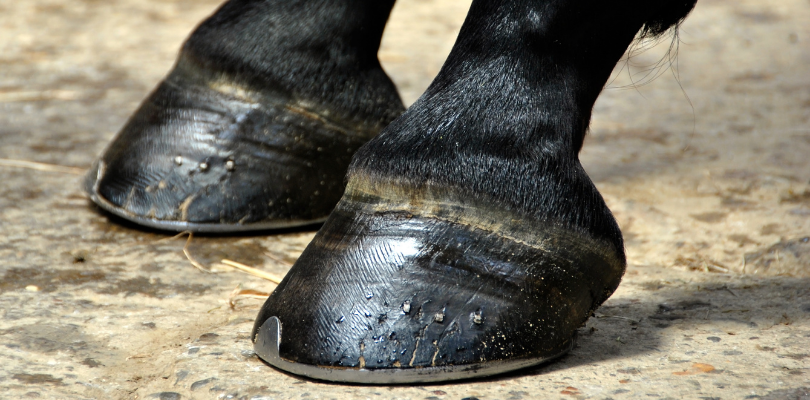This full-color, close-up photographic image, likely taken outdoors using natural light, features a pair of horse hooves on a hard brown surface speckled with gray rocks and a few bits of straw. The black hooves, reflecting the light, are fitted with silver metal shoes that have a semi-circular tip at the front and a metal band underneath. The image captures only the hooves and a few inches of the horse's short black-furred legs. The setting provides a rustic feel, possibly resembling a stable or an outdoor yard. The photograph's horizontally rectangular format emphasizes the detailed texture and sheen of the hooves and their shoes, without any text disrupting the scene.